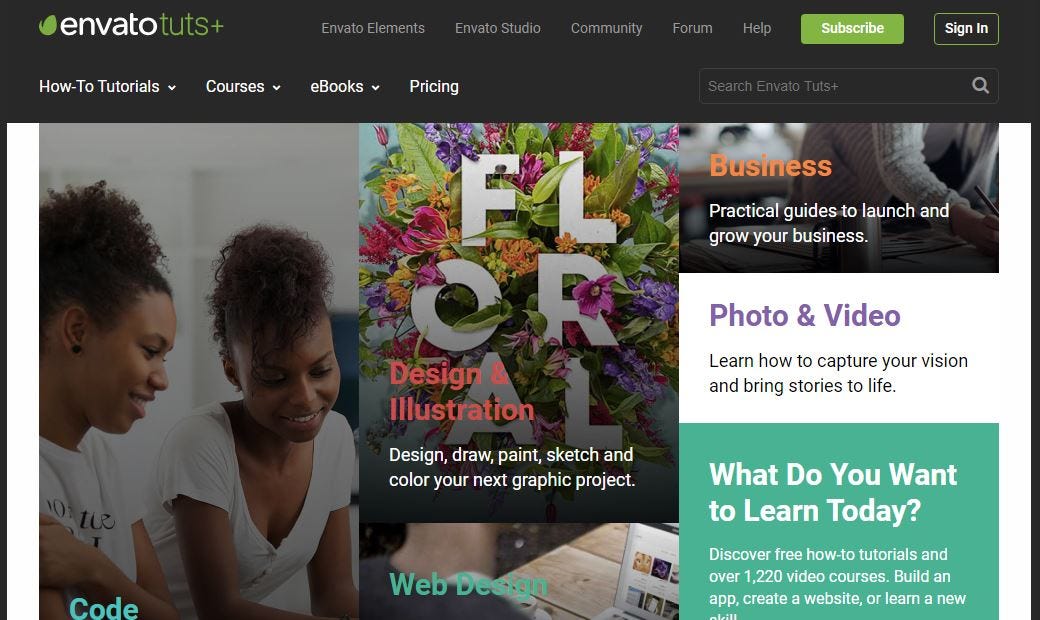The screenshot captures the homepage of the Envato Tuts+ website. At the top of the page, a navigation menu features links to Envato Elements, Envato Studio, Community, Forum, and Help, followed by a prominent green "Subscribe" button and a "Sign In" button. Just below this menu, there are options for how-to tutorials, courses, ebooks, and pricing. A search bar on the right, labeled "Search Envato Tuts+", includes a magnifying glass icon for easy navigation.

The main visual element of the page showcases two girls with curly hair tied into ponytails, both having dark skin. The girl on the left accessorizes with black earrings. Both are dressed in white t-shirts and appear to be gazing downwards intently. Surrounding them are several colorful keywords and categories. The word "Cold" is displayed in blue, "Web Design" in blue, "Design & Illustration" in red, "Business" in orange, and "Photo & Video" in purple. Adding to the page's vibrancy, there are decorative flowers in shades of pink, orange, and purple, accented with green leaves.